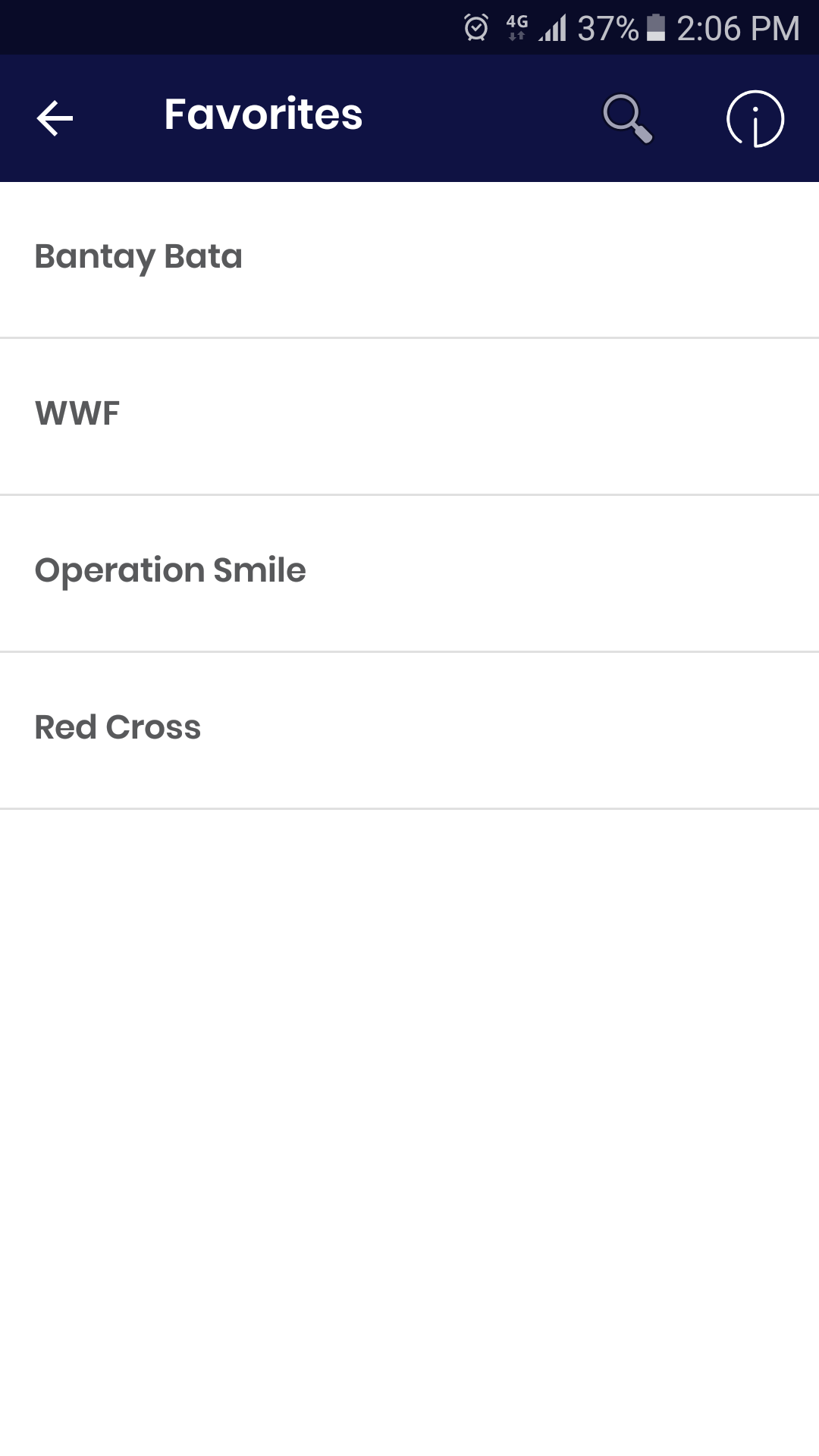In this image of a mobile app display, the screen showcases a list of charity organizations under the "Favorites" section. The interface is set against a navy blue border at the top, which frames the upper part of the app. In the upper right-hand corner, a white alarm clock icon indicates an alarm is set, while text displays a 4G mobile connection, a battery level of 37%, and the current time of 2:06 PM.

Just below the navy blue border, a white back arrow and the word "Favorites" in white lettering are prominently displayed. Adjacent to this is a search bar, accompanied by an information icon in the shape of an eye.

The main portion of the screen features a vertical list of favorite charities, separated by thin gray lines, effectively organizing the items in a bullet point style without actual bullet points. The listed charities are Banteay, Bataa, WWF, Operation Smile, and Red Cross, each clearly delineated for easy viewing and selection.